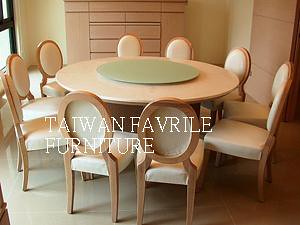This image is an advertisement for Taiwan Favrile Furniture, featuring a detailed display of a round, light wooden dining table surrounded by ten chairs. The table has a seafoam green Lazy Susan or mat at its center. Each chair has a wooden frame with a round, oval-shaped back, and they are upholstered with white cushions on both the seat and backrest. The room has off-white or beige walls with a grid-like pattern and light wood accents, possibly including shelves or drawers. The photograph shows the furniture on a wooden floor, contrasting with some descriptions suggesting linoleum. Additionally, there is a window in the upper left corner of the room which contributes to the light, airy atmosphere of the display. The text "Taiwan Favrile Furniture" is prominently featured across the center of the image, promoting the elegant and spacious yet somewhat compact arrangement of the dining set.